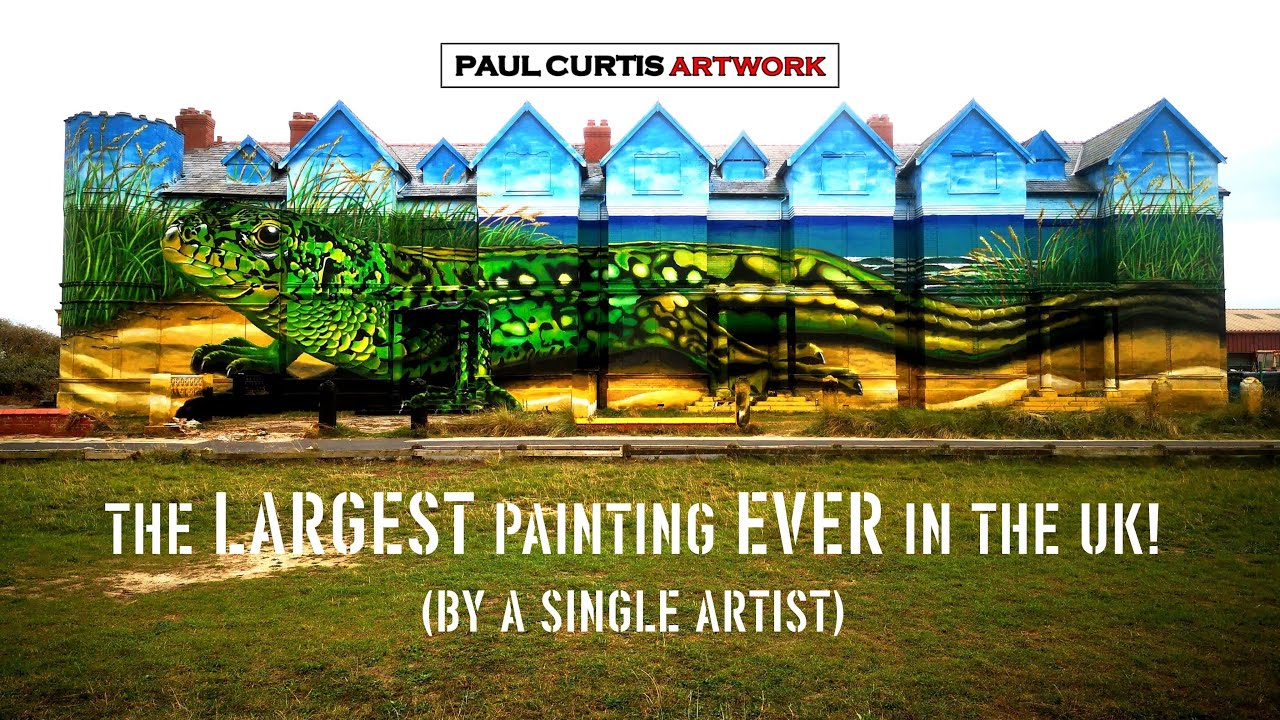This image showcases a significant artwork by Paul Curtis, as indicated by a label at the top of the image in black and red lettering stating "Paul Curtis Artworks." The scene depicts a row of approximately seven to nine connected townhouses that have been transformed into a sprawling mural. The mural features a sandy beach with an expansive, lifelike green iguana crawling across it. The upper sections of the houses are painted a calming blue, simulating an ocean or other body of water, complete with a blue sky and clouds, to create a seamless natural environment. A grassy field is visible at the bottom of the image, where white letters proclaim “The largest painting ever in the UK!” with a notation "(by a single artist)." This detailed painting integrates all components, creating an immersive, artistic landscape spread across the townhouses.